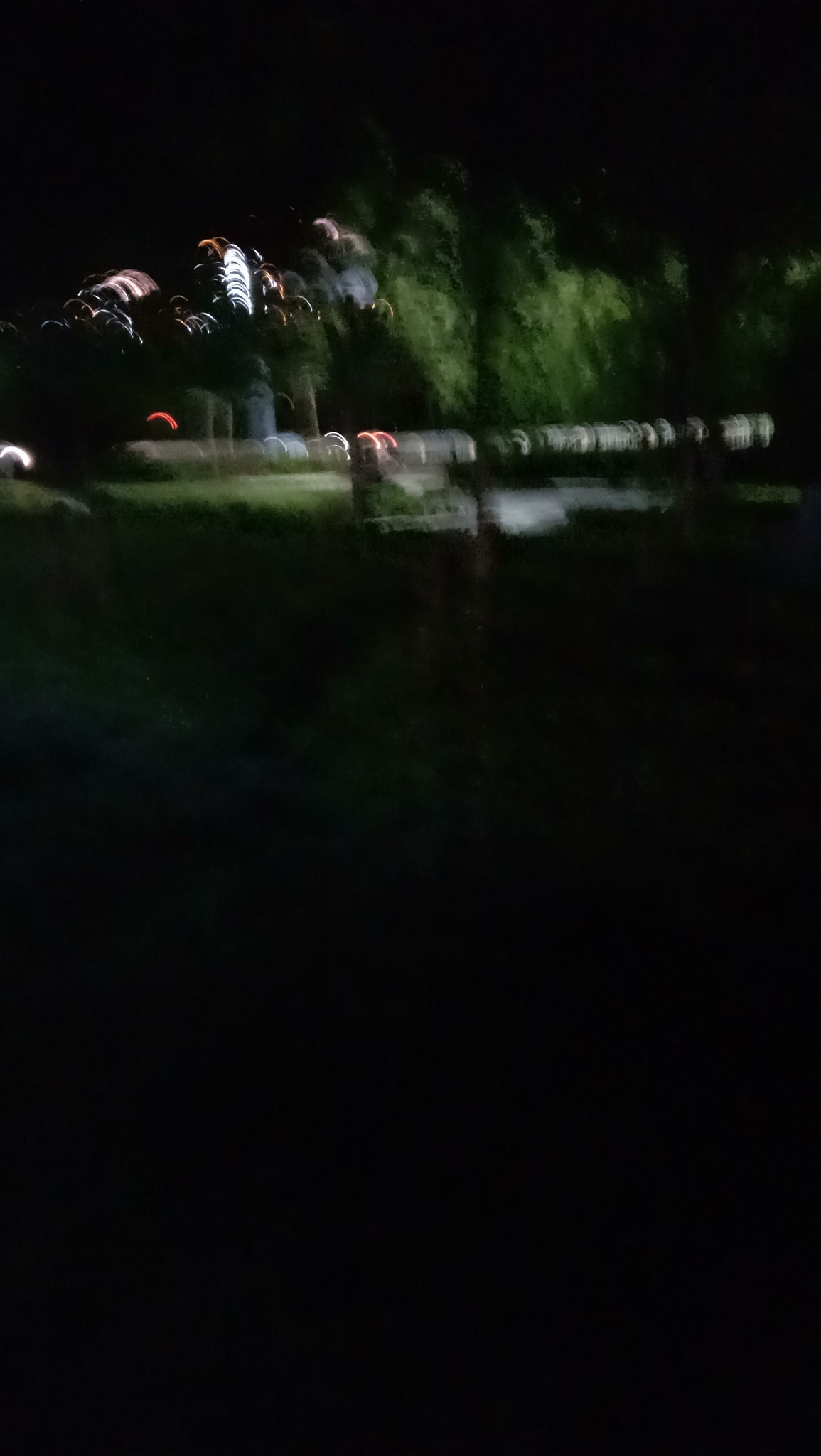The photograph in question is a highly blurred nighttime image, primarily dominated by darkness, covering around 80% of its entirety. The bottom and central sections of the image are almost completely black, suggesting it was taken during a drive by a vehicle, possibly capturing an unintended scene. Towards the upper quarter of the image, a faint and out-of-focus mixture of greenery, which could be trees or bushes, emerges. Interspersed within this vegetation, there are flashes of red, white, and yellow lights—likely from lampposts, vehicles, or other outdoor lighting sources. These lights create swirling patterns and a dome-like effect, coupled with some gray mist, adding to the indistinct and hazy appearance of the scene. The overall impression is of a nondescript nighttime view, obscured by poor lighting and motion blur.